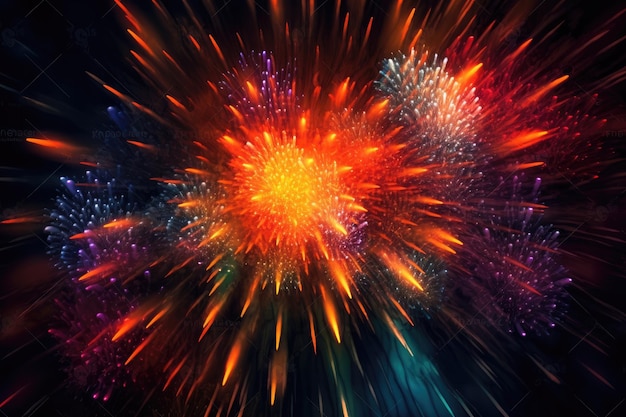This horizontal, rectangular photo captures the intense moment of a fireworks explosion against a black night sky. At the center of the image, a radiant burst of bright yellow blends into neon orange and darker shades of orange, creating a vivid focal point. Surrounding the central explosion are radiating fireworks with a spectrum of colors including yellow, blue, green, purple, red, and white, appearing as if they're coming directly towards the viewer. The edges of the fireworks are softer and more diffused compared to the crisp, detailed center. Smaller explosions of bright blue and white fireworks punctuate the periphery, adding layers of depth and a sense of motion to the scene. Overall, the photograph conveys the overwhelming and dynamic beauty of a large-scale fireworks display, filling almost the entire frame with vibrant, exploding colors and lights.